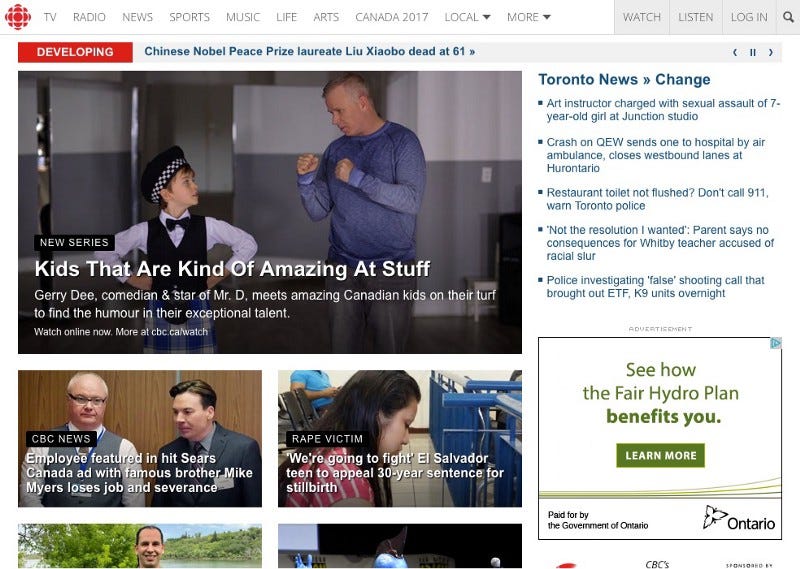Here is the cleaned up and detailed caption:

"The website homepage features a layout centered around a square logo with red accents and a circle in the middle, followed by the text 'TV.' To the right, a navigation bar includes tabs for TV, Radio, News, Sports, Music, Life, Arts, Canada 2017, and Local, with additional options in a pull-down menu. On the far right of the navigation bar are buttons for Watch, Listen, Log In, and a Search button depicted with a magnifying glass icon.

Beneath the navigation bar is a red rectangle labeled 'Developing' in white text. The main headline reads 'Chinese Nobel Peace Prize laureate Liu Xiaobo, dead at 61.' Below, there's an image featuring a child and a man with the caption 'New Series: Kids that are kind of amazing at stuff.' It describes that comedian and 'Mr. D' star Jerry D meets talented Canadian kids on their turf.

A second photograph displays two men with the caption, 'CBC News employee featured in hit Sears Canada ad with famous brother Mike Myers loses job and severance.' Adjacent to this is an image of a woman in a courtroom with the headline 'Rape victim in court. El Salvador teen to appeal 30-year sentence for stillbirth.'"